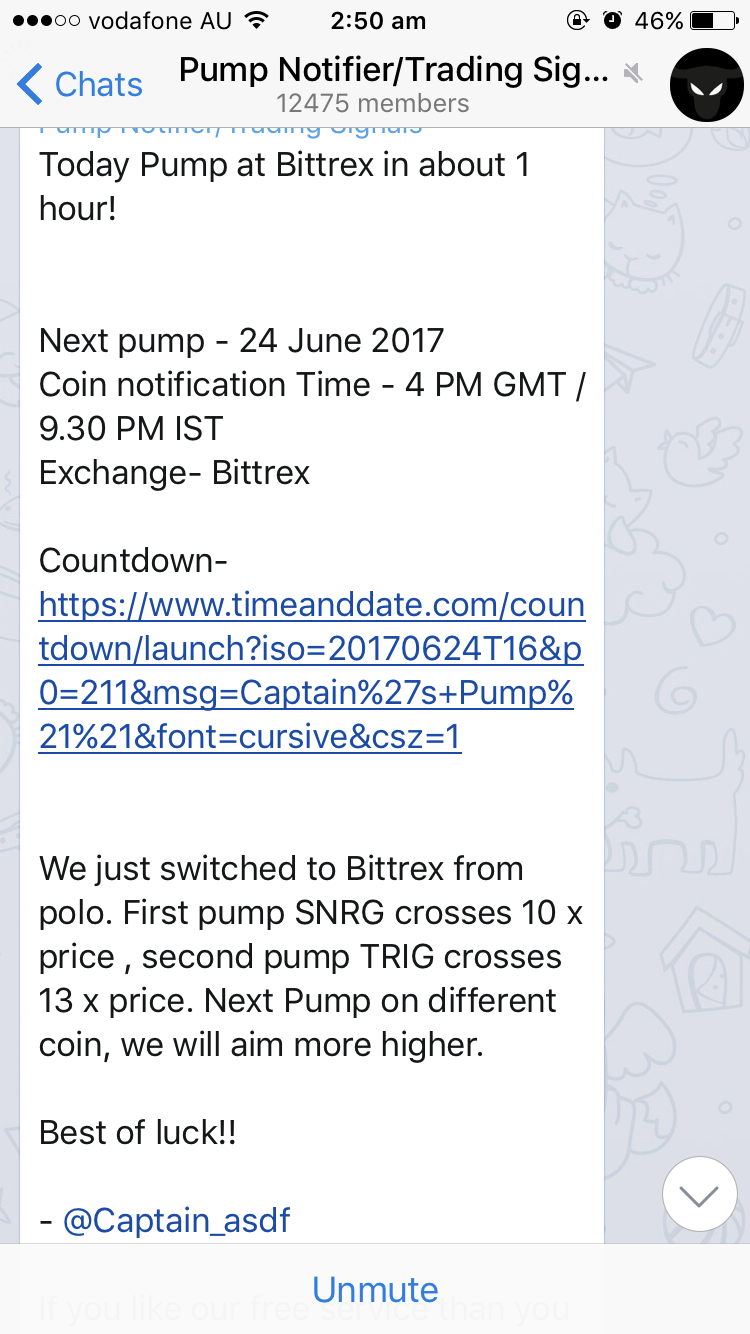This image is a cropped screenshot of a group chat on an Apple iPhone, showcasing a cryptocurrency pump notification group, identified at the top center as "Pump 9 Notifier/Trading Sig...". The full name is truncated. On the top left of the screen, there is a large arrow pointing left, and next to it, the word "Chats" is prominently displayed in large blue letters. The group has 12,475 members, indicated below the title, and a user profile photo on the far right that resembles a blacked-out bubble with two white eyes.

The body of the message within this group chat is contained within a blue background, adorned with pencil drawings of animals. To the left of the message is a large white chat box with an extensive text. The chat message starts with "Today pump at Bittrex in about one hour." It then details a further notification: "Next pump 24th June 2017 Coin Notification Time 4 p.m. GMT / 9:30 p.m. IST Exchange Bittrex". A link to a countdown is also provided. The message ends with a motivational "Best of luck" and is signed off with the handle "@CaptainASDF".

At the very bottom center of the screenshot, the word "Unmute," in large blue letters, indicates that the group chat is currently muted by the user. This screenshot shows a snapshot from a group likely dedicated to coordinating cryptocurrency pumps, similar to platforms like Robinhood or Bittrex.